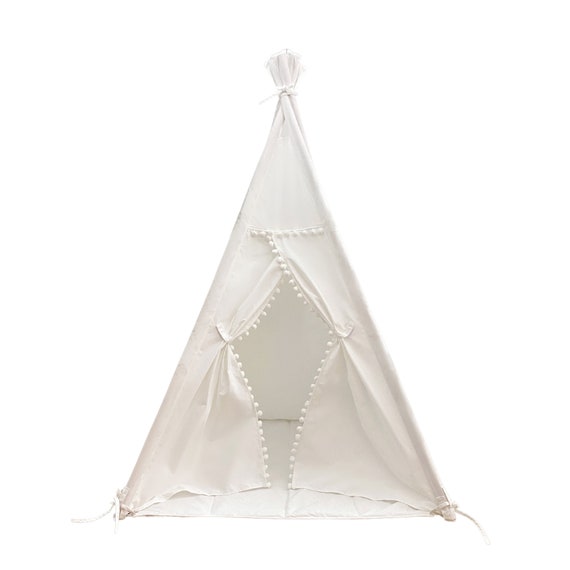The image shows a small, off-white, triangular pyramid-shaped tent, resembling a child-sized teepee, positioned centrally against a plain white background. The tent features an intricate design: its door, styled with interlocking elements, is held open widely in the middle and clips narrower at the top and bottom, creating a diamond-like opening. White pom-poms or beads adorn the door edges, enhancing its delicate appearance. The tent's fabric is sheer and possibly linen, with white strings or ropes tying it securely at the top and corners. The tent interior is completely empty, and the minimalistic background ensures there are no distractions from the tent's detailed structure.